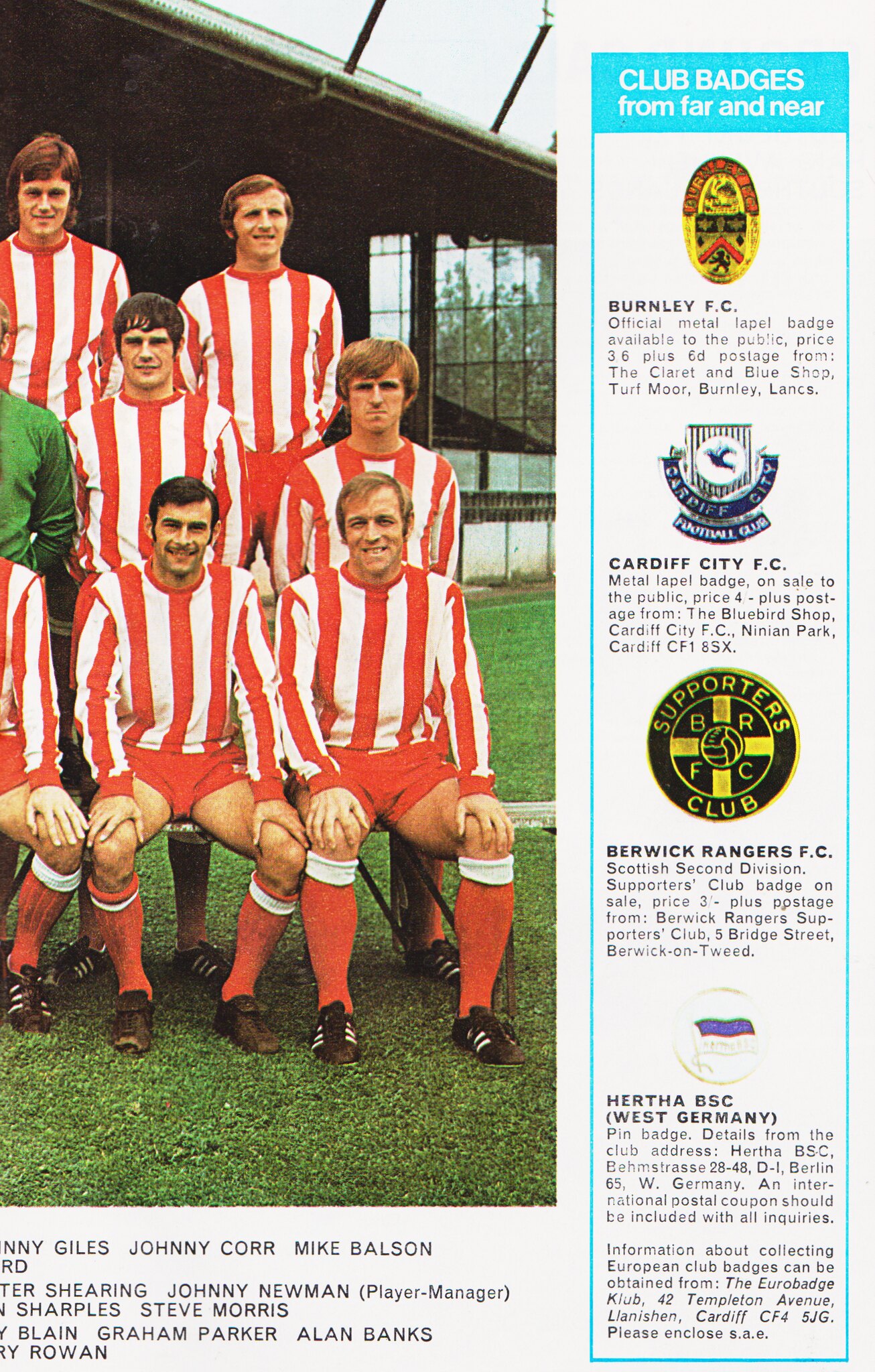The image appears to be a cropped page from a sports magazine or program booklet, depicting a partially visible team photo. The rectangular image is taller than it is wide and largely features an outdoor scene captured during the daytime. In the left two-thirds of the photo, several soccer players are dressed in matching red and white vertically striped long-sleeve shirts, red shorts, and red knee-high socks with white tops. 

The arrangement of the players includes two men sitting in the front row, two standing in the row behind them, and two more standing slightly off-center from the previous row. Additionally, a person wearing a green long-sleeve shirt – likely the coach – is partially visible on the left side of the image. The photograph is set against a grassy backdrop with a large building featuring big glass windows in the background, typical of a setting from the 1970s based on the hairstyles of the players. 

Beneath the photo, an incomplete list of names suggests an attempt to label the individuals. Some visible names are "N.N.Y. Giles, Johnny Core, Mike Balson" on one line, followed by partially visible text like "R.D" and "T.E.R Shearing, Johnny Newman, player manager," and further names such as "Sharples, Steve Morris, Blaine Graham Parker, Alan Banks, and R.Y. Rowan."

On the right side of the image, bordered in blue, a header reads "Club Badges, Far and Near." This section features several soccer club badges: a yellow and orangish-red oval badge labeled "Burnley FC," a blue and white badge for "Cardiff City FC," a black circle with a yellow cross for "Berwick Rangers FC Supporters," and a white circle with a purple and white flag insignia for "Hertha BSC West Germany." The section also includes text describing the sale of these badges, specifying prices and points of purchase like the Colourette and Blue Shop at Turfmoor, Burnley, or the Bluebird Shop at Ninian Park, Cardiff.